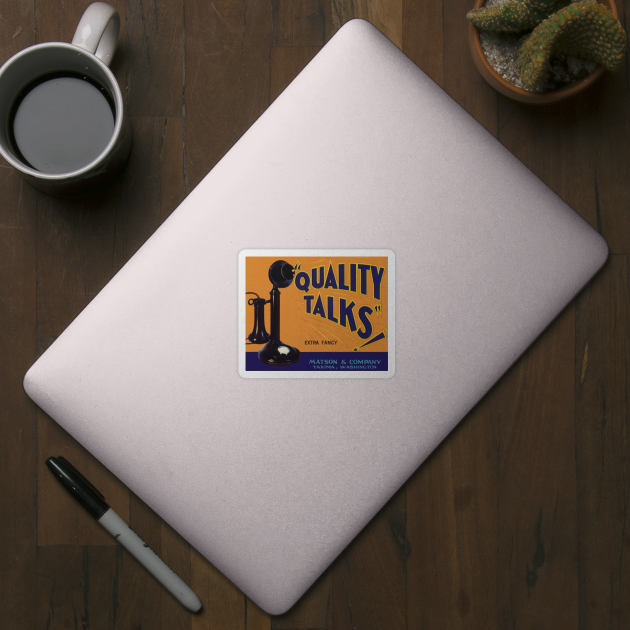In this top-down photo, a closed silver laptop sits on a dark brown wooden table. The laptop features a prominent sticker in the center, vividly colored in orange and blue, bearing the text "Quality Talks - Extra Fancy." The sticker displays an illustration of an old-fashioned, 1800s-style telephone with words appearing to come out of the speaker part. 

To the left of the laptop, a black-capped Sharpie rests diagonally, adding a touch of utility to the scene. On the upper left of the table, a white ceramic mug brimmed with coffee adds a homely feel to the arrangement. 

In the upper right corner, a small cactus plant, encased in a clay-colored pot filled with white rocky soil, adds a touch of greenery and life to the otherwise tech-focused setup. The wooden texture of the table underneath provides a warm and rustic background to the modern elements placed above it.